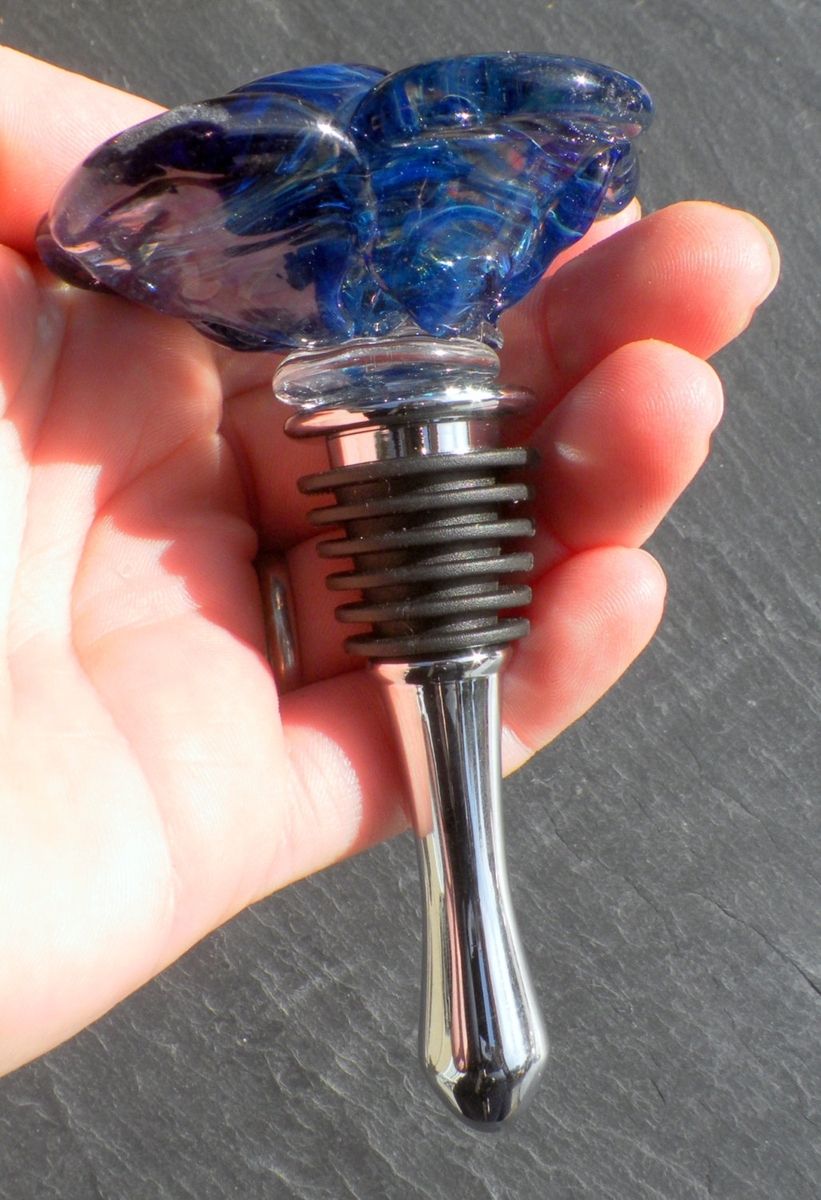In this detailed image, a person is holding a beautifully crafted wine stopper in their left hand, identifiable by the wedding band on their ring finger. The background showcases a plain gray slate, subtly lit by sunlight, which casts delicate shadows and highlights the object. The wine stopper features a tapered silver body with black rubber rings that ensure a snug fit into the wine bottle. A silver band separates the metal base from the ornamental glass top. Crowning the stopper is a clear glass ring supporting a striking blue glass flower, complete with graceful, curved petals and intricate swirls within the glass, resembling an artistic paperweight. The elegance of the blue glass flower, combined with the utilitarian design of the stopper, makes for a stunning and functional artifact that fits comfortably within the span of the handler's hand, from the index to the little finger.